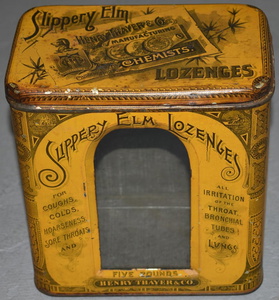The photograph depicts a vintage metal tin container for Slippery Elm Lozenges, likely from the early 20th century. The tin is mustard yellow in color and features some rust, indicating its age. The container is empty, revealing a gray interior through a cutout window on the front. The front label prominently displays "Slippery Elm Lozenges" in bold black lettering and lists the lozenges' purported benefits: relief for coughs, colds, hoarseness, sore throats, and irritation of the throat, bronchial tubes, and lungs. Below the viewing window, it indicates a weight of five pounds, suggesting it was intended for a large quantity of lozenges. The manufacturer is identified as Henry Thayer & Company. The top of the tin repeats the product name and features stylized stencil-like designs, a graphic of a lozenge pack, and the company's name. The worn appearance and classic design elements convey an antique quality.